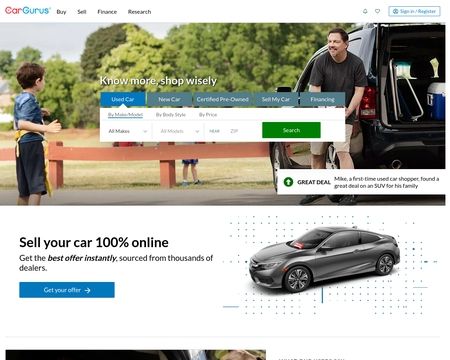This is a detailed screenshot from what appears to be the Car Gurus website, most likely displayed on a laptop. In the top left corner of the screen, the site’s logo is visible with "Car" written in red ink and "Gurus" spelled out as G-U-R-U-S in blue ink. The navigation menu is presented with four main categories: Buy, Sell, Finance, and Research. On the right side of the menu, there are two icons, though they are indistinguishable, accompanied by a sign-up/register bar.

The upper half of the screen features a photograph depicting a grown man standing next to a black SUV-type vehicle with its trunk open. In the trunk, there is a visible cooler. To the left of the man, a small male child can be seen with his feet visible in the background, standing near a brown fence. Behind the fence, a grassy field and some trees are visible, providing a scenic backdrop.

An inset bar in the foreground of the image offers five choices: Used Cars, New Cars, Certified Pre-Owned, Sell My Car, and Financing. The 'Used Cars' option is highlighted. One category within this section mentions 'Price,' though the complete details are not fully legible.

The bottom half of the screen includes a promotional banner stating, "Sell your car 100% online, get the best offer instantly, sourced from thousands of dealers," along with a blue clickable button labeled "Get Your Offer." Positioned near this text is an image of a gray sporty car with a dynamic blue dot design in the background, enhancing the visual appeal of the promotional offer.